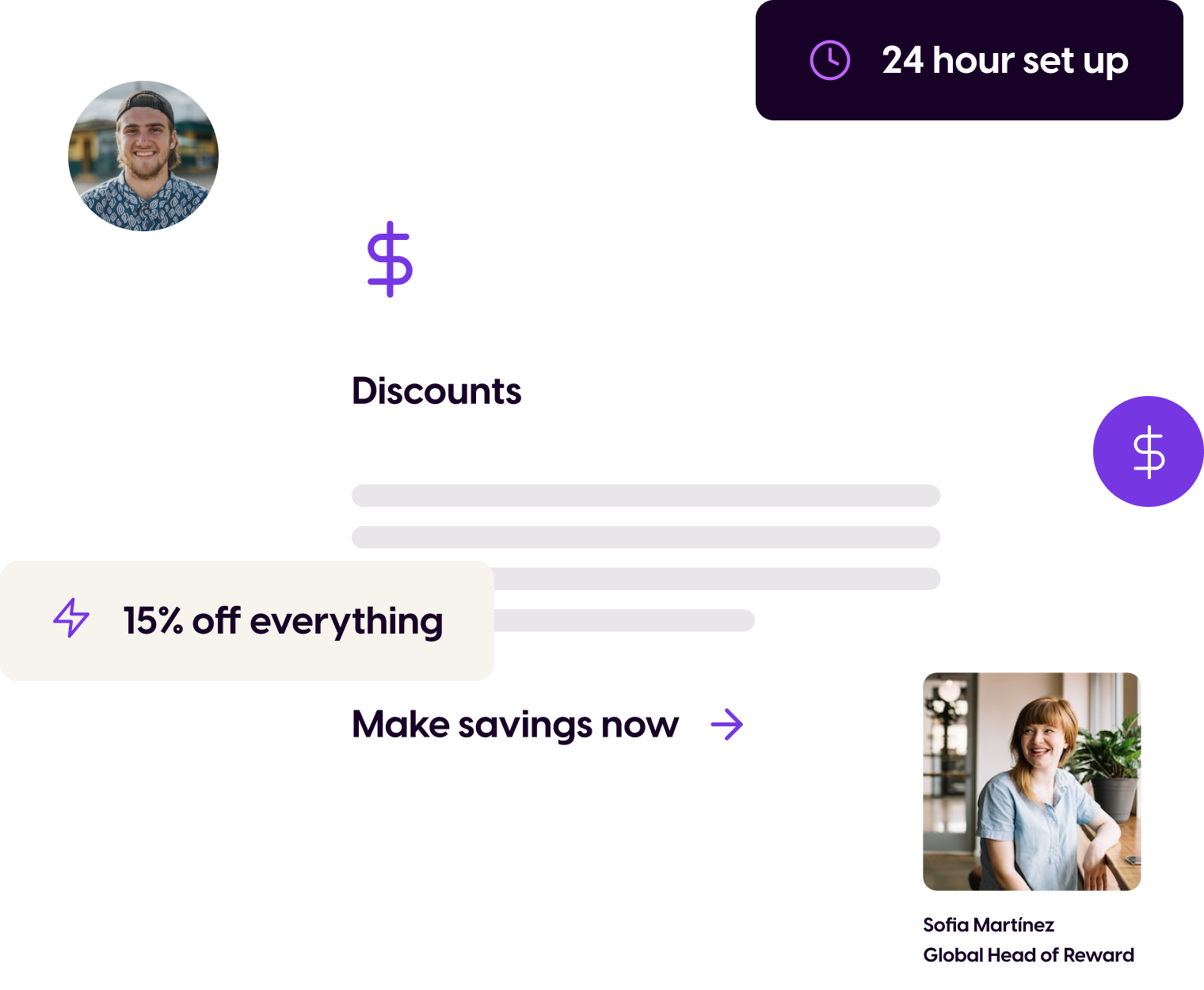The image is a square with a completely white background. In the upper right-hand corner, there's a horizontal rectangle with rounded edges, approximately four times wider than it is tall. At the center of this rectangle is a purple clock icon, followed by the text "24-hour setup" in white.

On the left side of the image, there is a profile picture of a smiling Caucasian man appearing to be around 30 years old. Directly below his picture, centered, is a purple dollar sign icon, followed by the text "discounts."

Below this, aligned to the left, there's another horizontal rectangle similar in dimensions to the first but in tan. Inside this rectangle, a purple lightning bolt icon is accompanied by the text "15% off everything" in black.

To the right of these elements, there are several horizontal graphic lines. Below these lines, centered, is bold black text reading "make savings now." A purple arrow points to the right from this text.

Finally, on the right side of the image, there is a picture of a smiling woman, identified as Sofia Martinez, with the title "Global Head of Reward" displayed below her photograph.